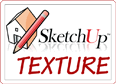This is an image of a close-up brick wall featuring a mix of red, brown, white, and gray bricks, some of which appear faded or sporadically placed. In the center of the image is a semi-transparent, oval-shaped watermark. This watermark contains an outline of a house with a pencil on top of it. Surrounding the house and pencil design, there are words written in a translucent, hard-to-read font, forming a circular pattern within the oval. The text includes a web address that partially reads "somethingclub.com" or "SketchUpTextureClub.com," although the exact words are difficult to decipher due to the pale, almost see-through style of the watermark.